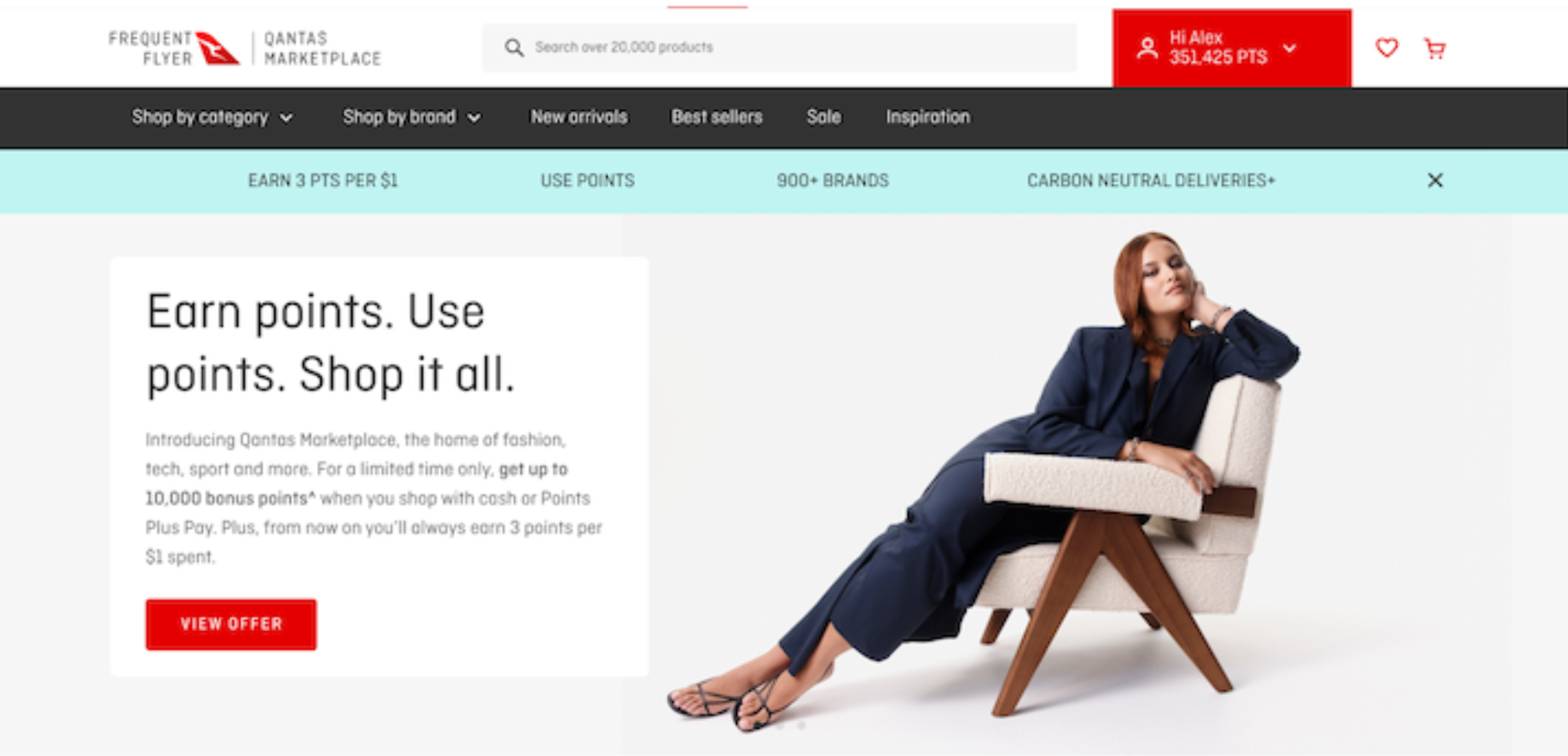This screenshot from a flight booking website showcases the user interface and features available to frequent flyer Alex. Logged in with an impressive balance of 351,425 points, Alex is navigating the Cantus marketplace, where points can be redeemed for products from over 900 brands. The website prominently features an image of a woman seated on a cream-colored recliner. Dressed entirely in navy blue, including her sandals, she leans back against the arm frame with a relaxed yet attentive demeanor, her bare ankles visible as she presumably enjoys the view. Adjacent to the image, a detailed box explains the process of using points within the marketplace.